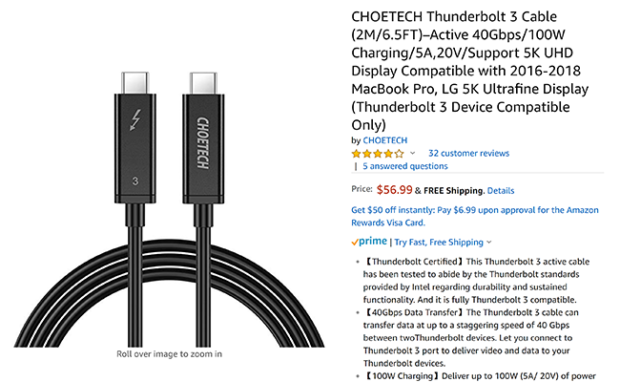The image depicts a product listing from Amazon, showcasing a CHOETECH Thunderbolt 3 cable. The left side of the image features a clean, white background with a clear, detailed photograph of the cable. The cable, black in color, displays silver connectors at both ends. The CHOETECH brand name is prominently visible. To the right, the product description is laid out clearly, identifying it as a "CHOETECH Thunderbolt 3 Cable, Active 40 Gbps Charging, Support 5K." Further down, the product has been rated four stars based on 32 customer reviews. The listing also indicates availability for Amazon Prime members, highlighting the benefit of free shipping. Additional details about the cable's specifications and features are provided beneath the reviews and Prime shipping badge.